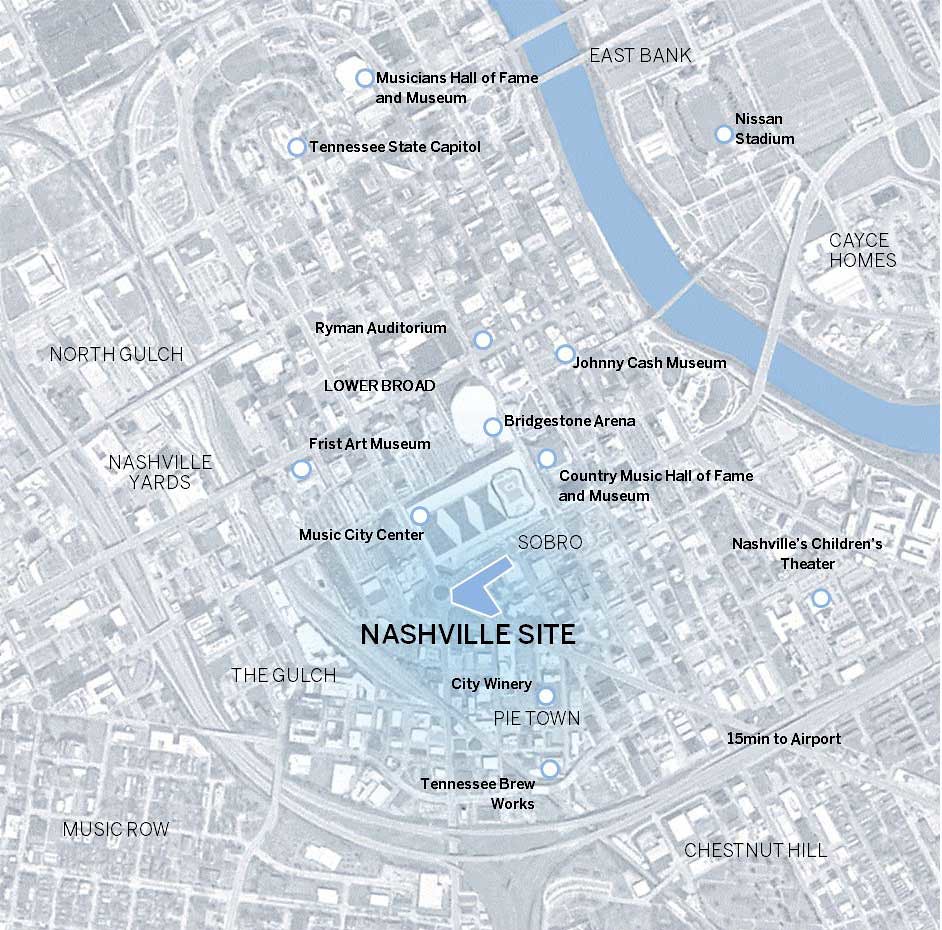The image is a detailed bird's-eye view map of Nashville, predominantly displayed in grayscale with blue marking the waterways, capturing various significant landmarks and locales. Centrally, the map highlights the "Nashville site," pinpointing notable locations such as East Bank, Nissan Stadium, Musicians Hall of Fame and Museum, and the Tennessee State Capitol. Also included are cultural and entertainment venues like the Ryman Auditorium, Lower Broadway, Bridgestone Arena, Johnny Cash Museum, Country Music Hall of Fame and Museum, Music Center, Nashville Children's Theater, Chestnut Hill, and Pie Town City Winery. Notably, the map omits roadways but meticulously labels the buildings and structures, offering a comprehensive layout of this central Nashville area.